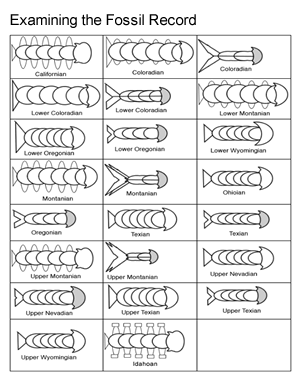The image is a detailed black-and-white chart titled "Examining the Fossil Record," appearing to be from a magazine or book. It consists of eight horizontal rows, each containing three labeled columns, totaling 24 individual illustrations. Each cell in the chart features crudely drawn, pen-like sketches of fossilized creatures, resembling centipedes or segmented worms, with circles that connect via half-circles and tail-like structures.

The labels at the top of the chart sequence the fossil types according to various American regions, such as Californian, Coloradian, Montanian, and Texian, among others. Some regions have variations like "Lower Coloradian" and "Upper Nevadian," indicating stratigraphic or temporal differences within the same geographical location. Specific labels include Californian, Coloradian, Lower Coloradian, Lower Montanian, Lower Oregonian, Lower Wyomingian, Montanian, Chioan (likely a typo for Ohioan), Oregonian, Texian, Upper Montanian, Upper Nevadian, Upper Texian, Upper Wyomingian, and Idahoian. The chart documents the state-specific attributes of these fossils, possibly showing their completeness, body structure, and distinguishing features from different regions across the United States.